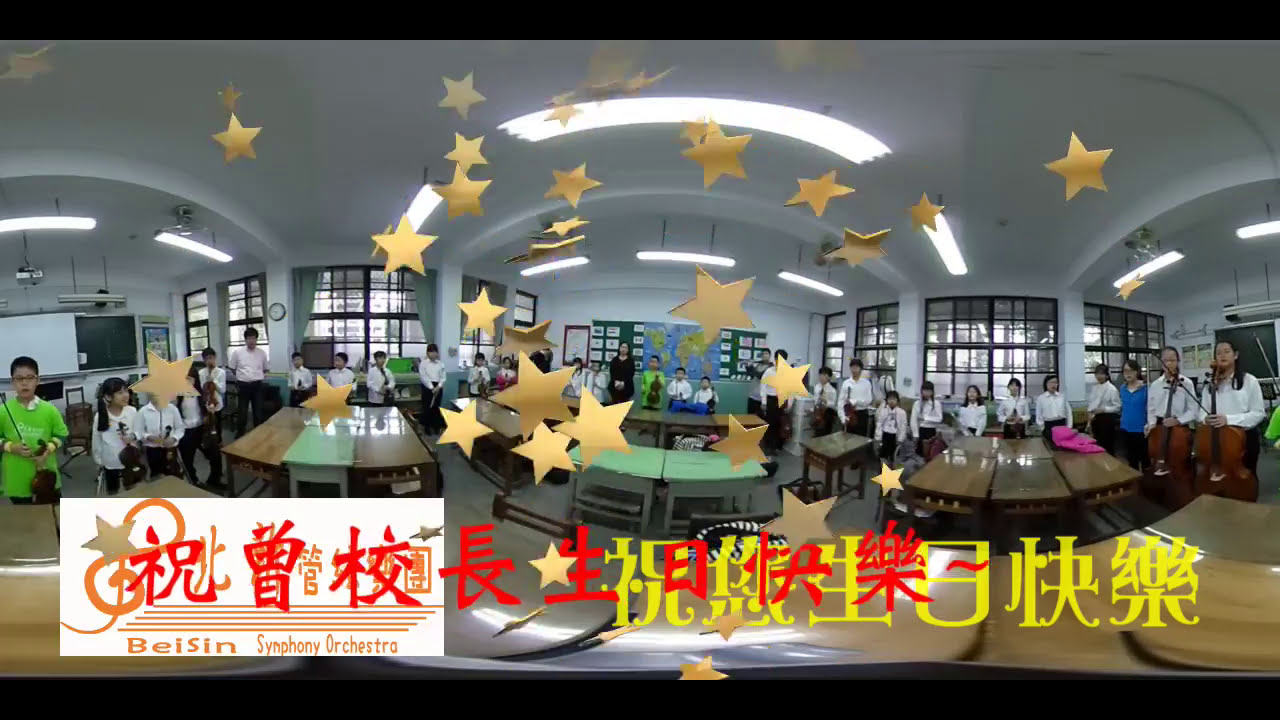The image is a panoramic photo of a Chinese classroom, overlaid with numerous shiny, 3D gold stars. Along the bottom of the image, there's a white rectangle containing red and yellow Chinese text and the logo "Bae Sin Symphony Orchestra." Below the text, part of the background appears blurred and rounded, giving a soft, bulbous aesthetic. 

The students, dressed in white shirts and black pants, stand along the walls where large windows provide ample light. They are holding violins and larger string instruments, like cellos, of light brown wood in one hand and bows in the other. Some teachers, wearing black, are interspersed among the students. The classroom features a white ceiling with three distinct white arches. The overall scene reflects a formal, organized setting, blending the cultural essence with musical elements.